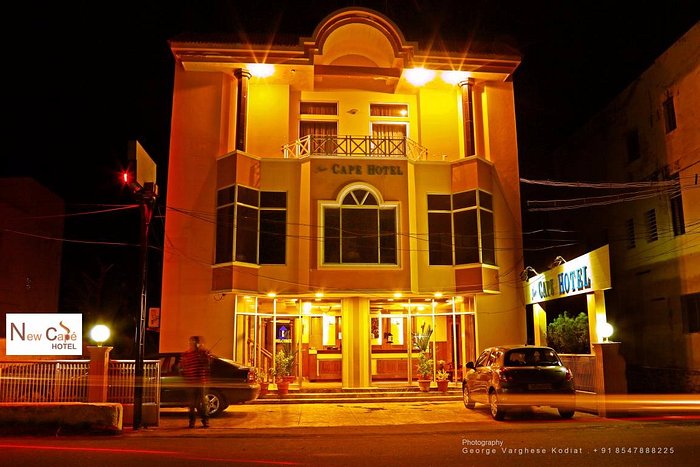This photograph captures the New Cape Hotel at night, a three-story building glowing with a warm, golden hue against a black sky. The hotel's facade, characterized by Art Deco elements and a simple, rectangular architecture, is prominently lit. A white sign on the lower left reads "New Cape Hotel," while a larger, illuminated sign on the right side spells out "Cape Hotel," facing the street. The ground floor of the hotel is enclosed in glass, revealing the front desk area with potted plants and a well-lit lobby. The middle floor features several dark windows, indicative of unused or unlit rooms, and the top floor boasts a small balcony with glass doors, lit by lights under the eaves. In the foreground, there's a brown road or parking area with two cars—one parked directly in front of the hotel and another parked diagonally. A blurred figure stands near one of these cars. The scene is framed by silhouettes of buildings and power lines in the background, giving a sense of an urban setting. There's also an inscription on the right side providing the photographer's contact details: "George Varghese Kodiat +91 85478882255 or 225."